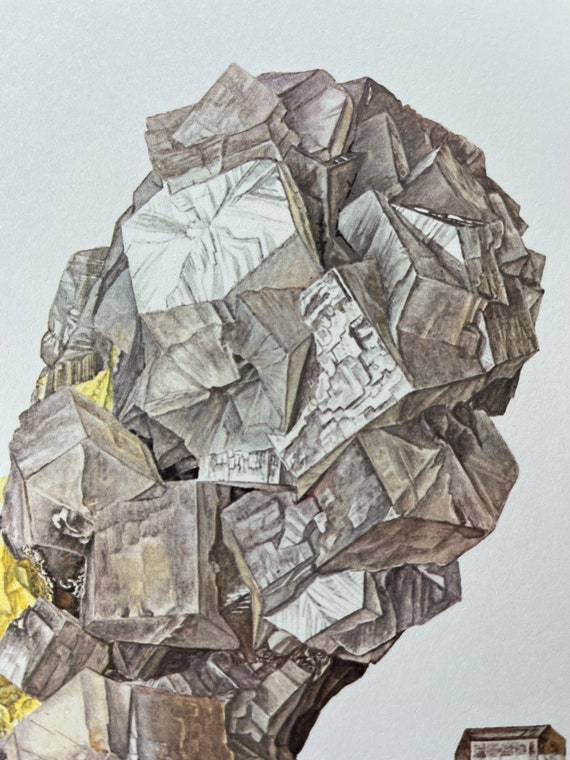This piece appears to be an abstract illustration in a portrait layout, where the top and bottom sides of the image are shorter than the sides. The image features a striking geometric mass extending diagonally from the lower left corner to the upper right corner. This mass is composed of fragmented and angular shapes resembling metallic boulders, shards, and cubes. The intricate formation has varied textures and is predominantly rendered in shades of gray, white, and black. There are subtle pops of yellow along the left-hand side and occasional accents of gold at the very bottom left. The background is a soft off-blue or light gray color, adding depth to the overall composition. The image is devoid of any people or text, focusing entirely on the abstract structure that evokes impressions of fragmented buildings or a mineral column, reminiscent of scenes from the movie "Inception" where city landscapes fold and stretch surrealistically towards the sky.